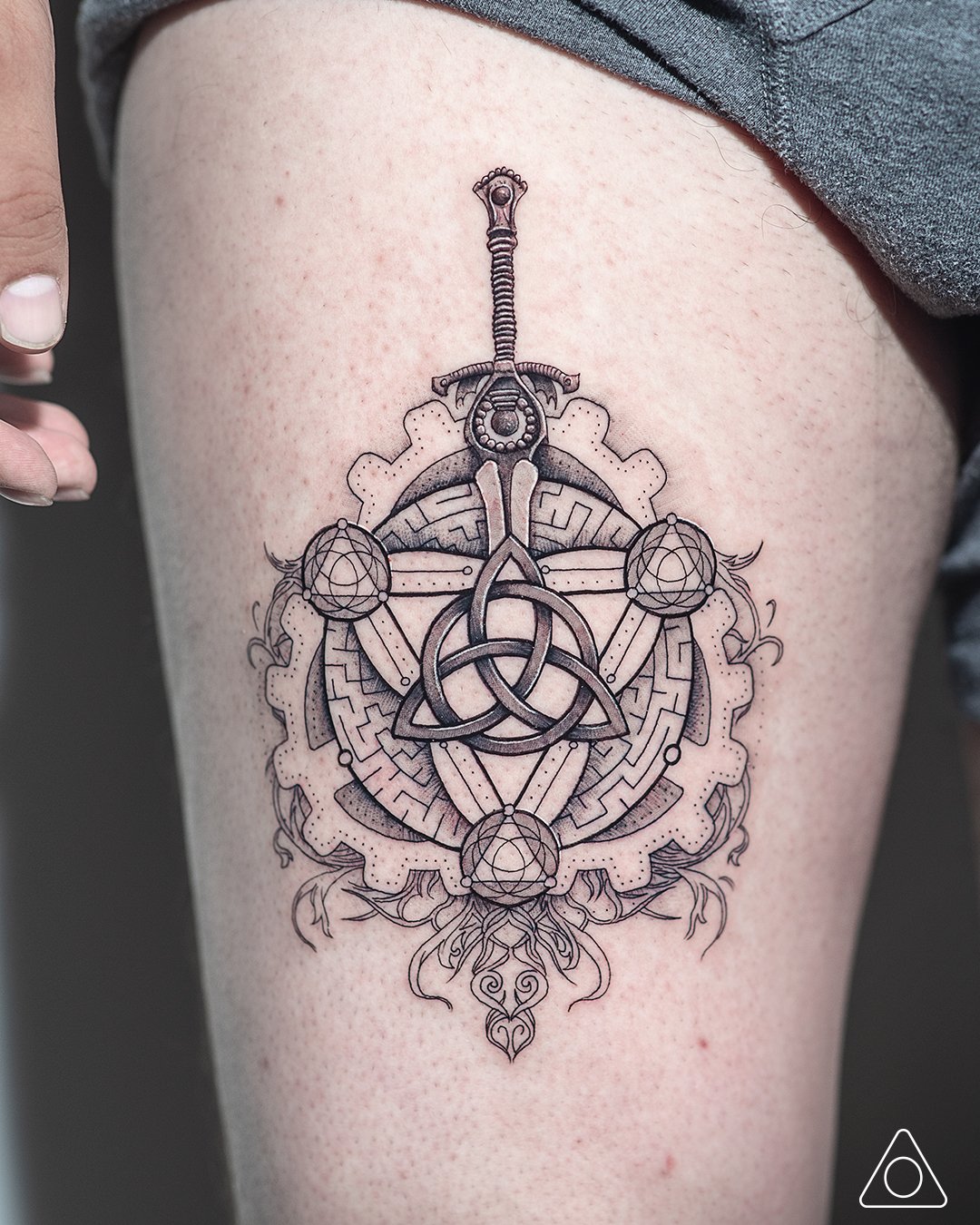This color photograph, in portrait orientation, captures a detailed black line art tattoo on the upper thigh of a Caucasian individual with light pink skin, suggesting the tattoo is freshly applied. The person is wearing dark gray terry shorts, and their left hand hangs naturally beside their leg. The intricate tattoo, situated from just above the panty line to just above the knee on their right thigh, features a medieval-inspired design evocative of "Lord of the Rings" or ancient gladiator heraldry. The centerpiece is a circular configuration with three intersecting gears, over which lies the handle of a saber or dagger extending from the top. Within the circular formation is a maze-like center, overlaid by a triangular shape with a Celtic knot at its core. The tattoo incorporates a complex network of intertwining rings and leaves, forming additional triangles within a larger circle. Decorative scroll features adorn the bottom and sides, enhancing the elaborate design. The background of the image is black, making the white triangle with a white circle in the bottom right corner stand out distinctly.